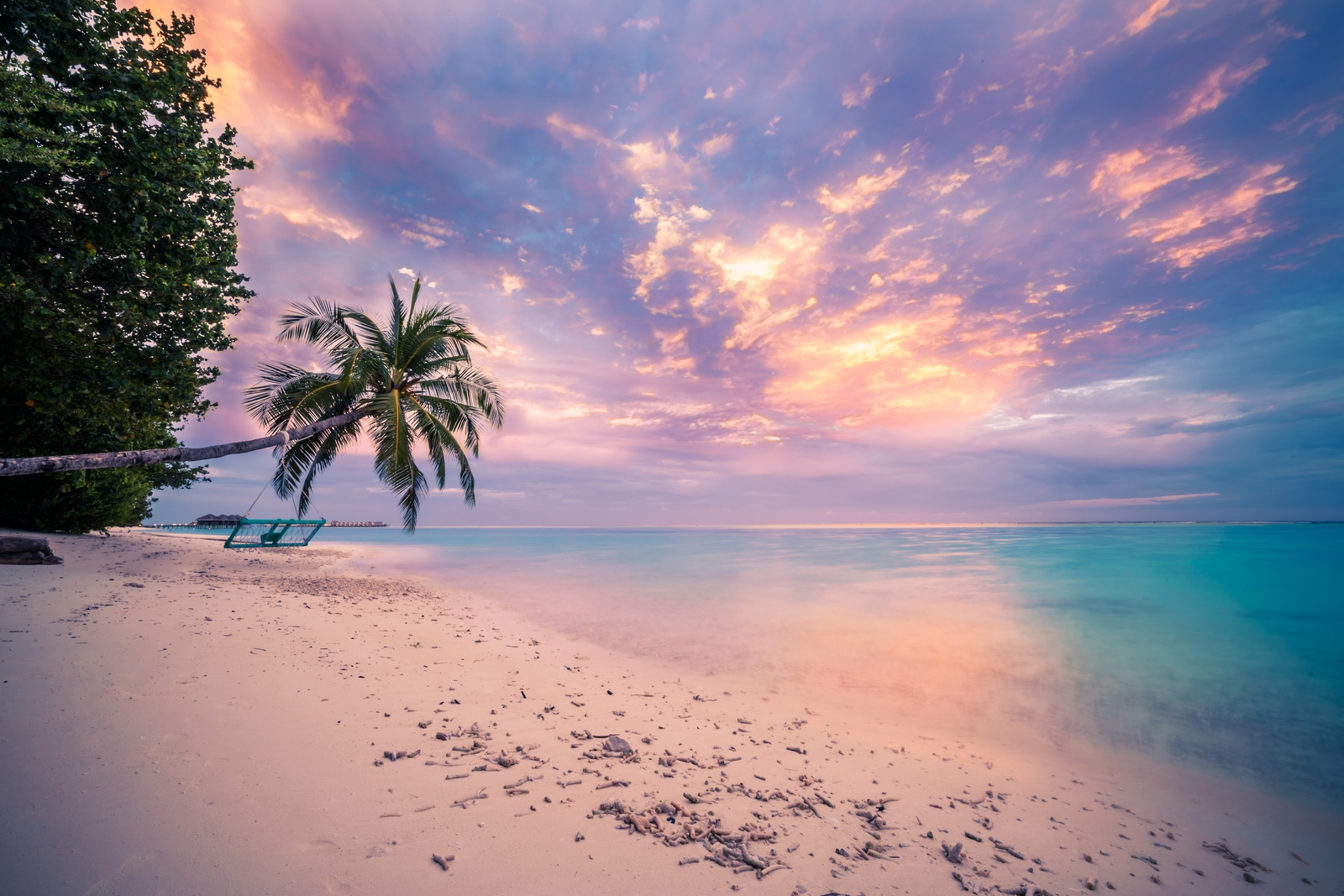The photograph captures a stunning tropical beach scene viewed from the shore, emphasizing a beautiful sunset with a colorful, cloudy sky in shades of purple, orange, and hints of yellow. Dominating the left side of the image is a large, leafy green bush and an intriguing, horizontally tilted palm tree extending over the beach and into the ocean. From the trunk of this palm tree, a white rope swing hangs invitingly. The shoreline, covered in beach sand dotted with small plants, stretches across the bottom of the frame. The serene ocean water transitions through muted pastel hues, starting with pink near the beach, blending into green, and finally into blue further out. In the distance, structures on stilts can be seen, adding a touch of rustic charm to the horizon. This striking photograph captures the vibrant yet tranquil essence of a tropical sunset beach scene.